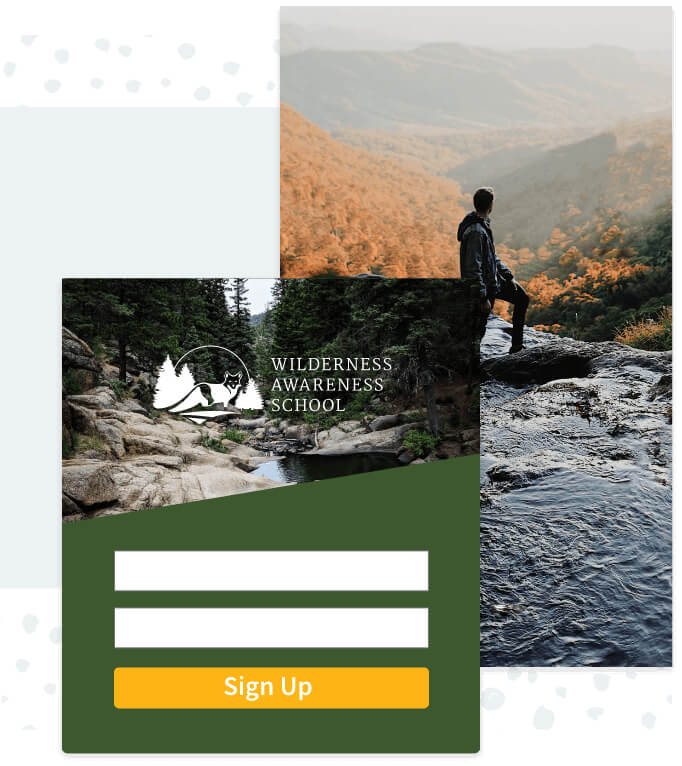The image is divided into two distinct sections, bordered by white margins at the top and bottom, with light gray, abstract splotches and dots filling the background. The primary focus on the right side is a color photograph of a man standing on two rocks in a river. He faces away from the camera, gazing out towards a valley that extends into distant mountains. Superimposed in the bottom left corner is another square image that overlaps part of the main photograph. This smaller image features a river scene surrounded by wilderness, complete with river rocks and trees. Positioned over this scene is white text that reads "Wilderness Awareness School." Below this, the image transitions into a dark green background segmented into three long rectangular boxes. The top two boxes are white and empty, while the bottom box is yellow with white text that states "Signed Up."